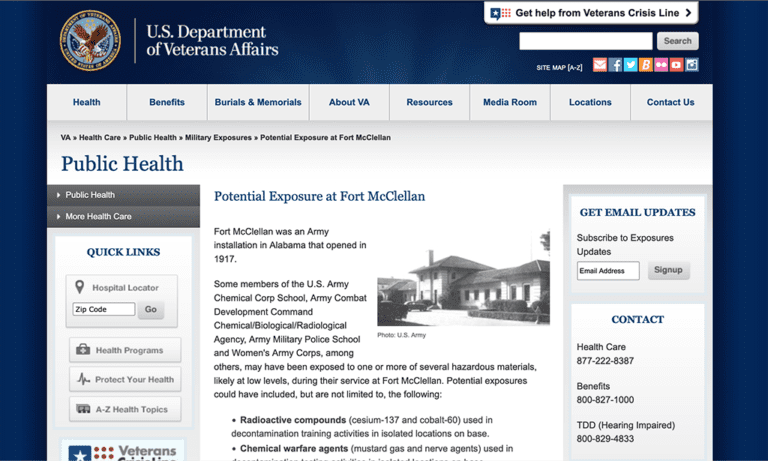The screenshot depicts a webpage from the U.S. Department of Veterans Affairs. In the upper left corner, the official logo featuring an eagle and the U.S. flag is prominently displayed. Adjacent to it, the upper right section includes a white rectangular banner with black text that reads, “Get help from Veterans Crisis Line,” followed by a right-pointing arrow icon and a search bar.

Below the header, there is a blue navigation bar offering various clickable categories such as Health Benefits, Burials and Memorials, About VA, Resources, Media Room, Locations, and Contact Us. The main content area headlines "Public Health" and features an article titled “Potential Exposure at Fort McClellan.” This article addresses potential chemical and radioactive exposure risks faced by individuals at Fort McClellan. Accompanying the text, a black-and-white photograph of Fort McClellan is positioned slightly to the right of center.

In the bottom right corner, a contact information box lists various phone numbers available for further inquiries.